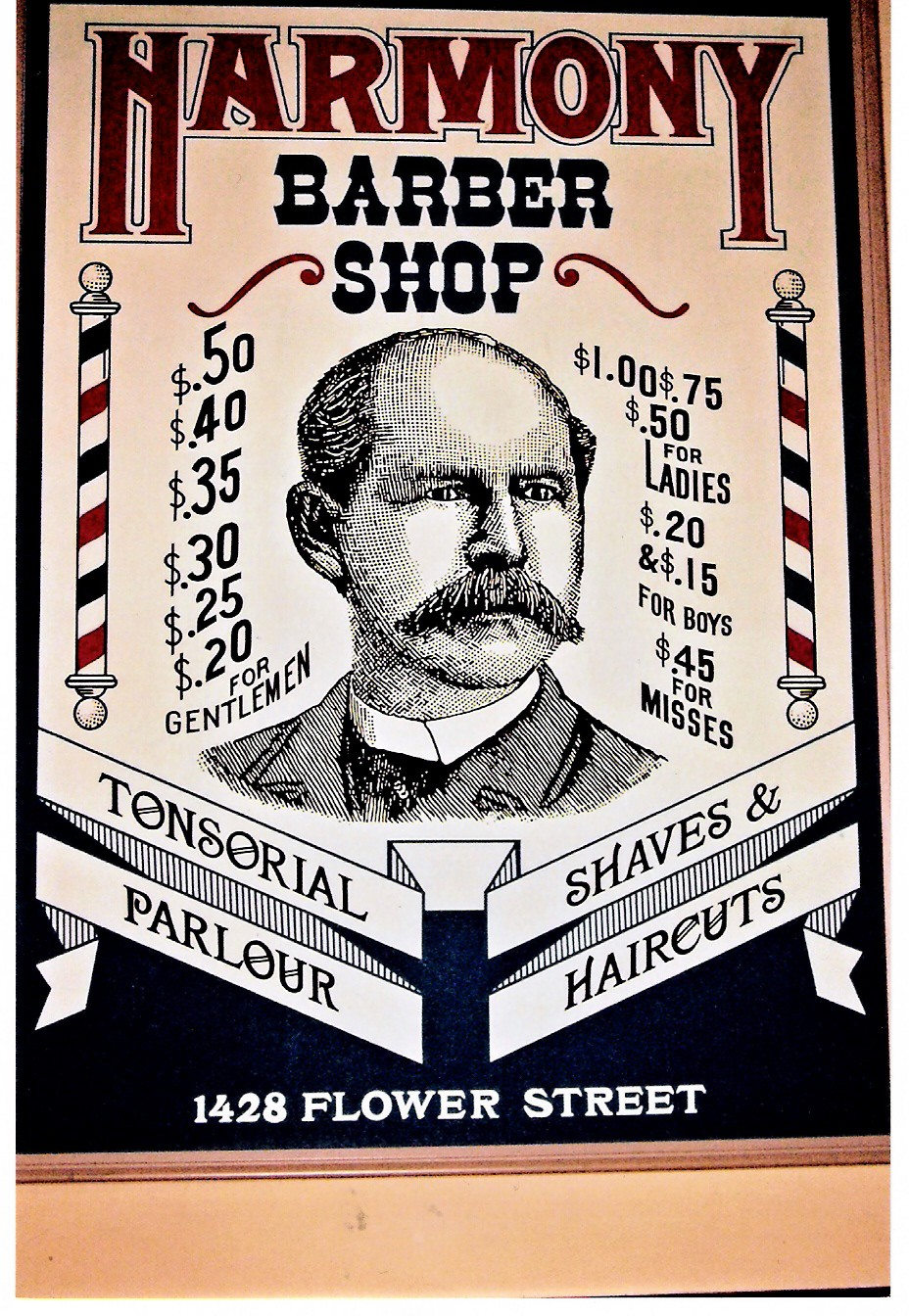This image is an old-fashioned advertisement poster for the Harmony Barber Shop, located at 1428 Flower Street. The poster features a vintage aesthetic with plain, old-timey fonts reminiscent of early newspaper prints. At the top, the name "Harmony Barber Shop" is prominently displayed. In the center of the poster is a detailed drawing of a man with a receding hairline and a large, thick mustache, wearing a stiff-collared white shirt and a coat.

On the left side of the poster, prices for men's services are listed, ranging from 20 to 50 cents, with options detailed at 50 cents, 40 cents, 35 cents, 30 cents, 25 cents, and 20 cents. On the right side, the prices for women's services are shown, ranging from 50 cents to 1 dollar. Additional prices include 15 and 20 cents for boys and 45 cents for the missus. 

The bottom portion of the poster features the words "tonsorial parlor" on the left and "shaves and haircuts" on the right, arranged in diagonal boxes beneath the man's image, emphasizing the variety of grooming services offered.